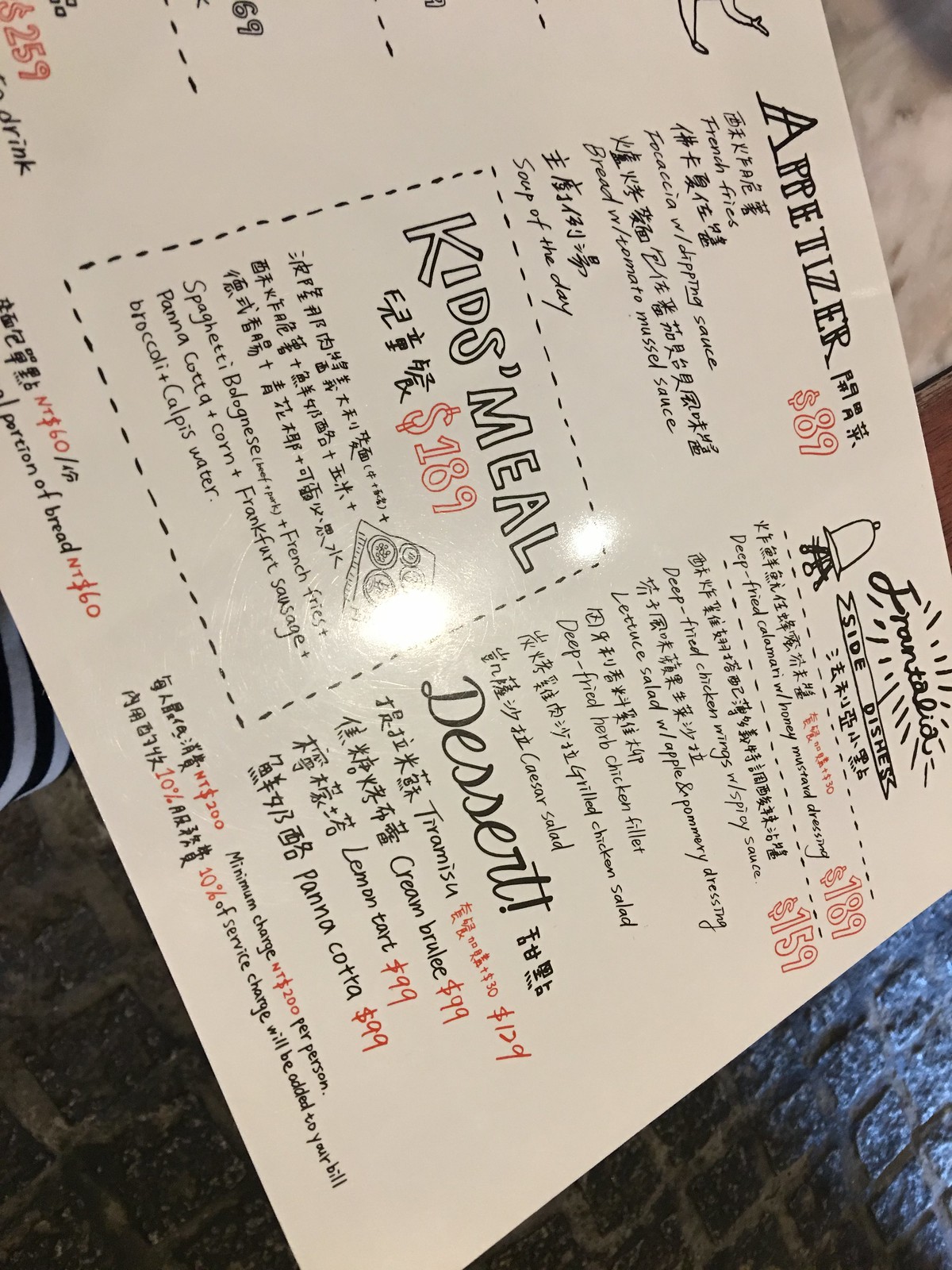The image captures a portrait-oriented photo of a menu, which diagonally spans from the top left to the bottom right of the frame. It's noteworthy that about two-thirds of the menu is visible and it appears on white laminated paper. The middle column prominently features the heading "Appetizer" written in a stylish handwritten font, with additional characters inked in black beside it. Below this heading, the listed items include:

- French Fries
- Focaccia with Dipping Sauce
- Bread with Tomato Mussel Sauce
- Soup of the Day

Each item is accompanied by written characters directly above it.

Towards the lower part of the middle column, there is a segmented box outlined with broken lines, containing the label "Kid's Meal" in bold bubble letters. Beneath "Kid's Meal" is a sequence of black characters followed by the price, written in red: $189. The meal includes a detailed list of:

- Spaghetti Bolognese (Beef and Pork)
- French Fries
- Panna Cotta
- Corn
- Frankfurt Sausage
- Broccoli
- Cowpea Water

In the right column of the menu, several categories and items are listed. Under the "Frontalia" heading, the following items appear:

- Deep Fried Calamari with Honey Mustard Dressing ($189 in red ink)
- Deep Fried Chicken Wings with Spicy Sauce ($159)
- Lettuce Salad with Apple Pommery Dressing
- Deep Fried Herb Chicken Filet
- Grilled Chicken Salad
- Caesar Salad

Farther down, under the "Dessert" section, the following sweets are listed:

- Tiramisu (with red characters and a price of $129)
- Creme Brulee ($99)
- Lemon Tart ($99)
- Panna Cotta ($99)

The arrangement of text and pricing effectively guides the reader through the menu's offerings while maintaining a clear and organized presentation.